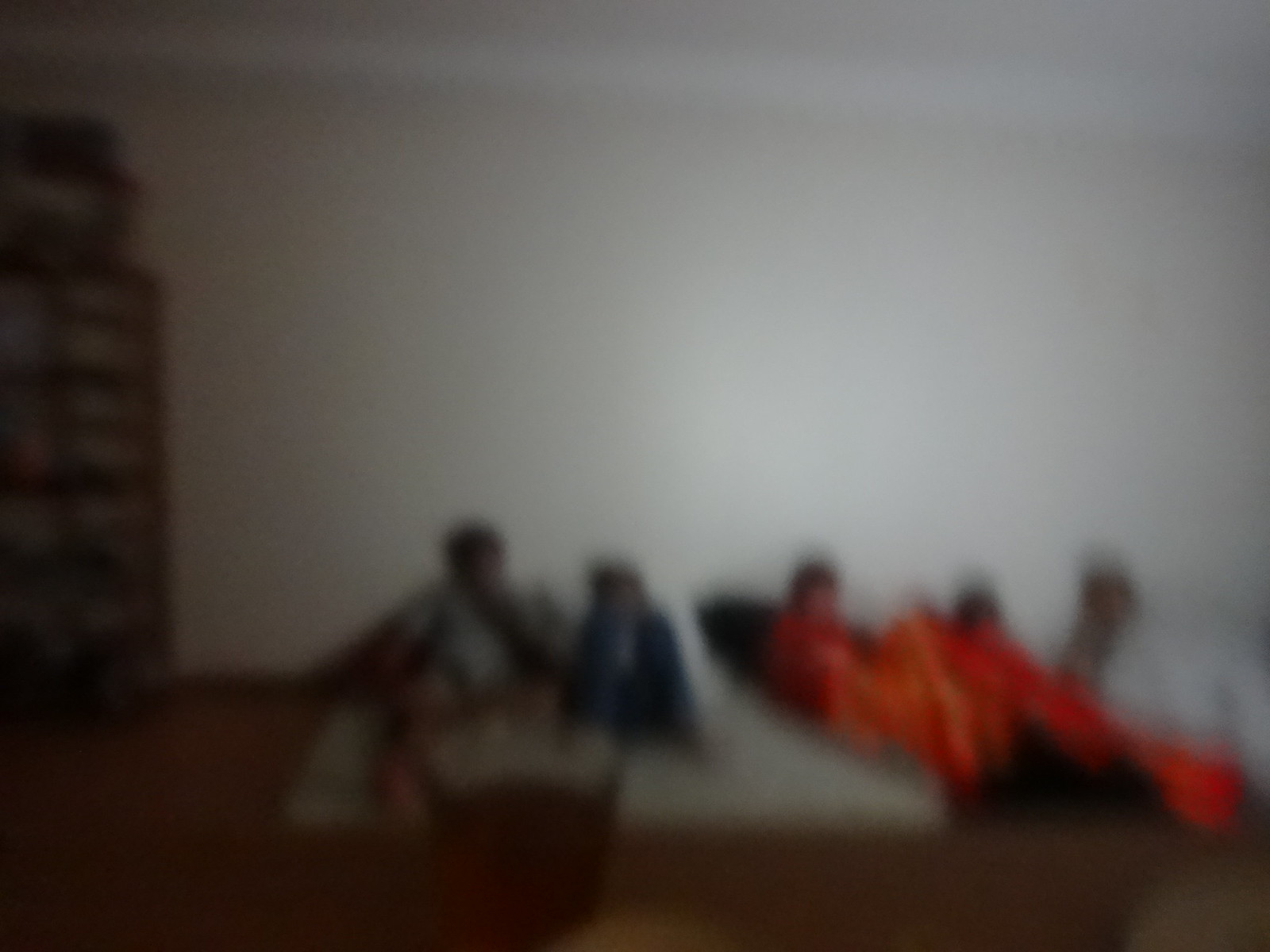A group of five individuals is seated on the floor, each covered with blankets or possibly using pillows, creating a cozy atmosphere. They are sitting on mats, one of which is white and the other black. A woven basket is placed nearby, and a bookshelf stands against the stark white wall, adding a touch of homeliness to the space. The individuals' faces are blurred, making it hard to distinguish their features, suggesting an emphasis on privacy. The setting appears to be an uncluttered living room, furnished with typical bedroom comforts such as blankets and soft seating, indicating they might be spending an extended period in this serene environment.